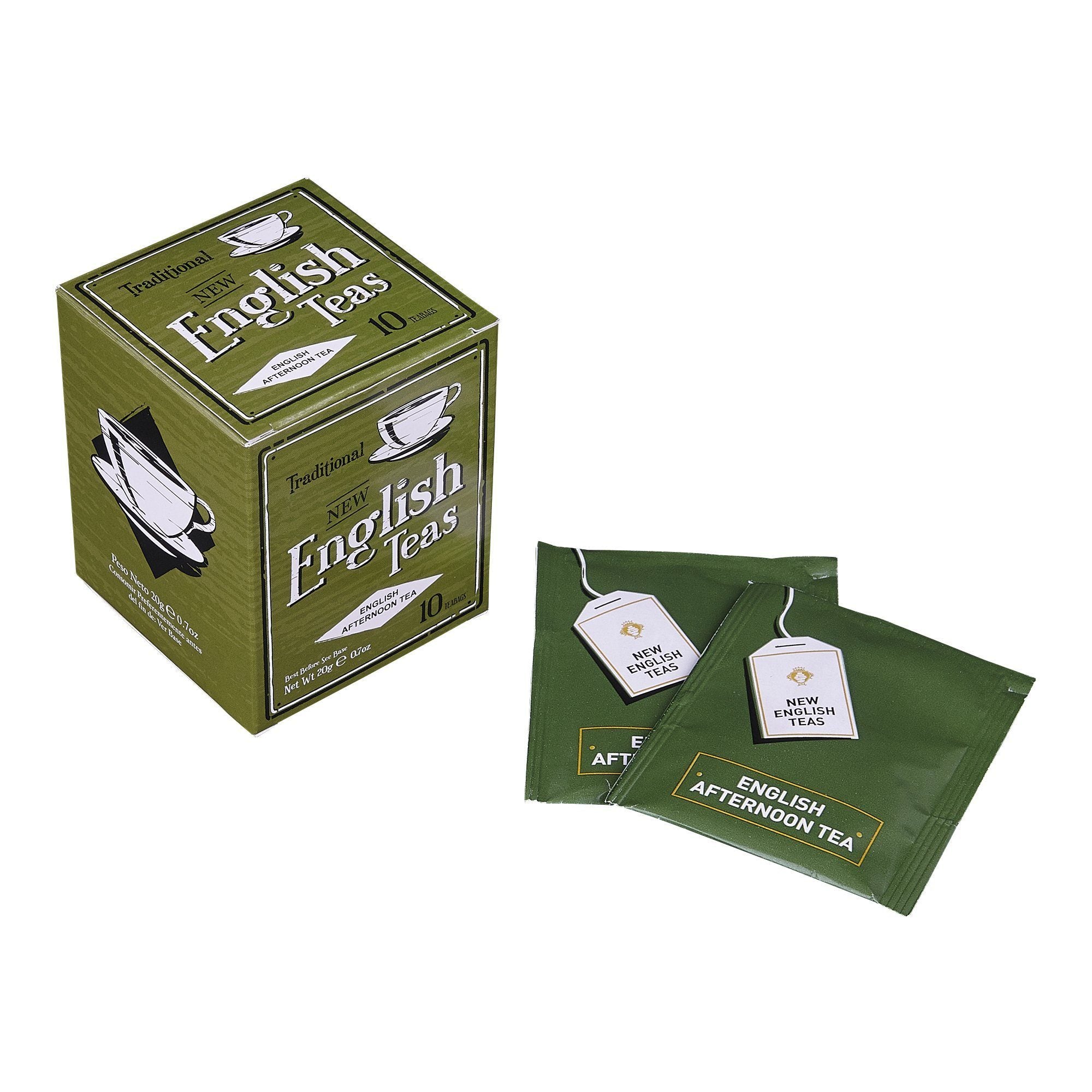The image depicts a green, cube-shaped box of traditional New English Teas' English Afternoon Tea. The light forest green packaging features a black diamond on the left with a white teacup and saucer illustration. On the front, the text "traditional" is displayed in black above "NEW" in uppercase black letters, and "English Teas" in superimposed white text. Below this, within a white diamond with black text, it reads "English Afternoon Tea." The box is labeled with a net weight of 20 grams (7 ounces) and indicates it contains 10 tea bags. This design is mirrored at the top of the box. Additionally, it showcases a similar white teacup and saucer on the right, with two dark green tea bags placed beside the box. These tea bags have a tag at the top that reads "New English Teas" and are marked "English Afternoon Tea" in a rectangular gold box at the bottom.